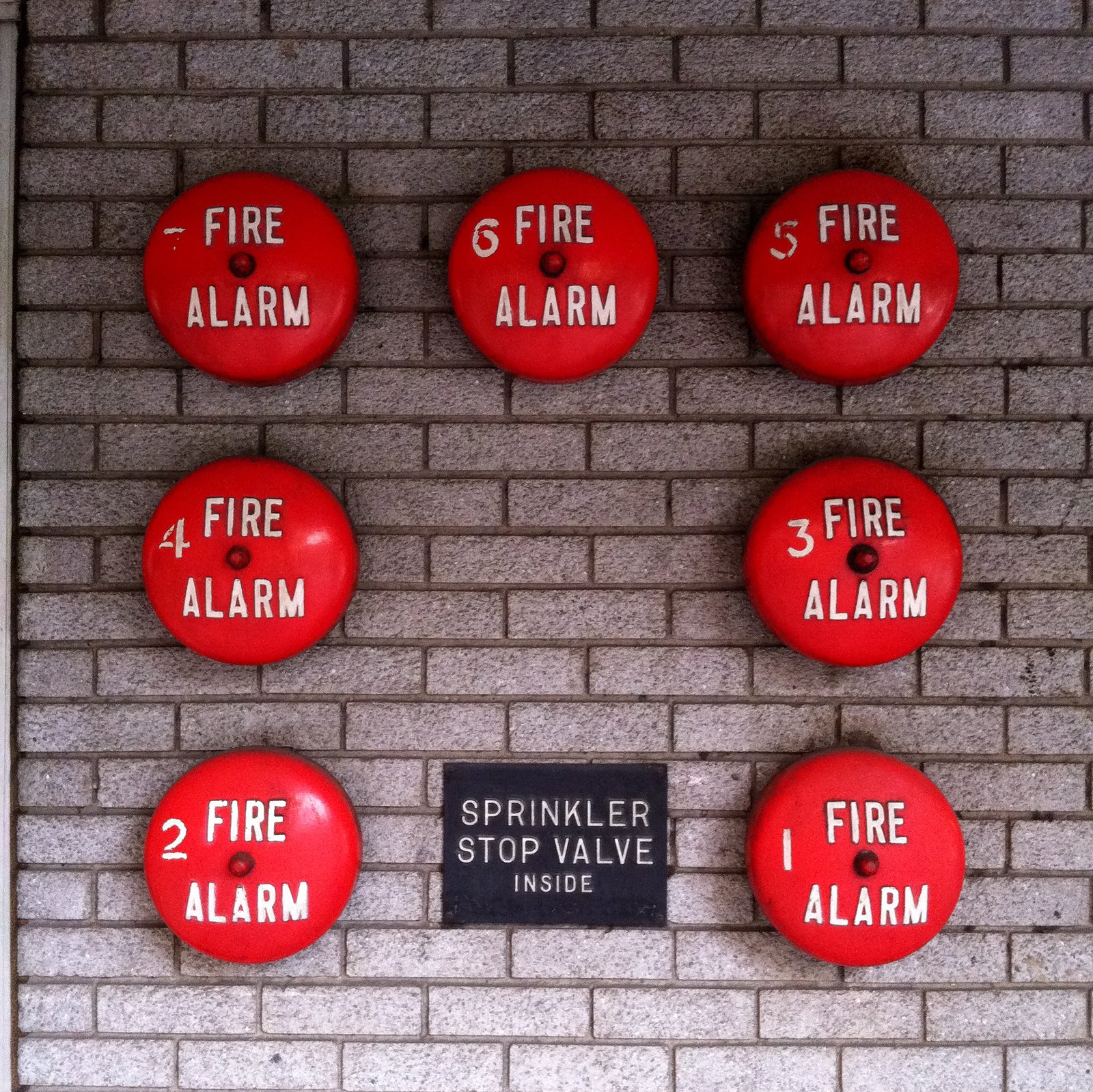This image showcases a segment of a gray brick wall with a notable speckling of white. Prominently mounted on the wall are seven red circular fire alarm bells, each labeled with the words "FIRE ALARM" and numbers one through seven. The bells are arranged to form a square-like shape: three bells across the top, two in the middle row, and two at the bottom row. Embedded at the center of this arrangement, where the seventh bell in the middle row would be, is a black plaque that states "SPRINKLER STOP VALVE INSIDE" in bold white capital letters. The left-hand bells are numbered 4 and 6, while the right-hand bells display numbers 3 and 1. The top row of alarms is labeled 5 (left), 6 (center), and 7 (right). The bottom row mirrors the top row in distribution, with the alarms numbered 2 (left) and 1 (right). The orderly presentation, combined with the distinctive numbering and central safety plaque, adds a systematic and alerting aspect to the structural design.